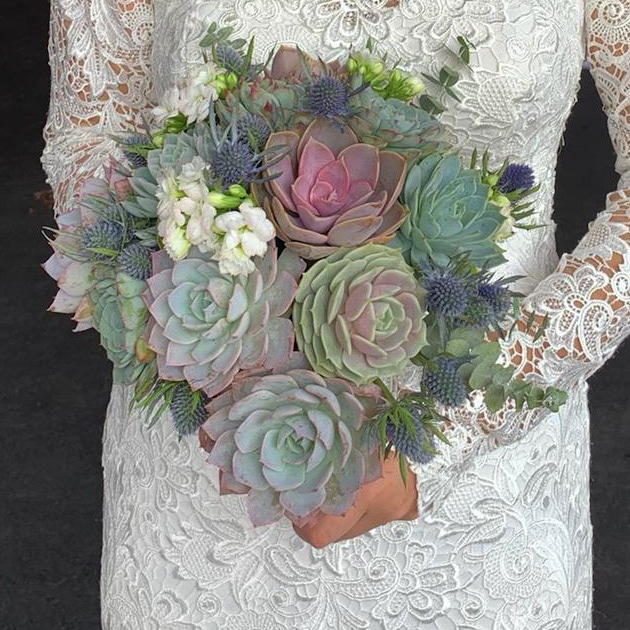In this photograph, a bride is elegantly posed against a dark backdrop, highlighting her stunning white wedding dress that is intricately adorned with lace. The dress features prominent floral lace designs, with long, see-through sleeves that extend nearly to her hands, revealing glimpses of her tan skin through the delicate fabric. The bodice and sleeves are a satiny, shiny crochet lace, which adds a luxurious texture to the ensemble. The bride holds a large, vibrant bouquet of succulents in front of her, consisting of a variety of colors including pink, purple, white, green, and hints of red. The succulents, some resembling blackberries, are joined by pieces of eucalyptus and other floral elements, creating a striking and colorful contrast to her all-white attire. The bouquet's unique, felt-like texture and pastel hues lend a whimsical, almost surreal quality to the arrangement, suggesting it might be a crafted piece rather than natural blooms. The shot captures the bride from just below her shoulders to mid-thigh, centered to emphasize both her intricate lace dress and the abundant, eye-catching bouquet she cradles between her arms.